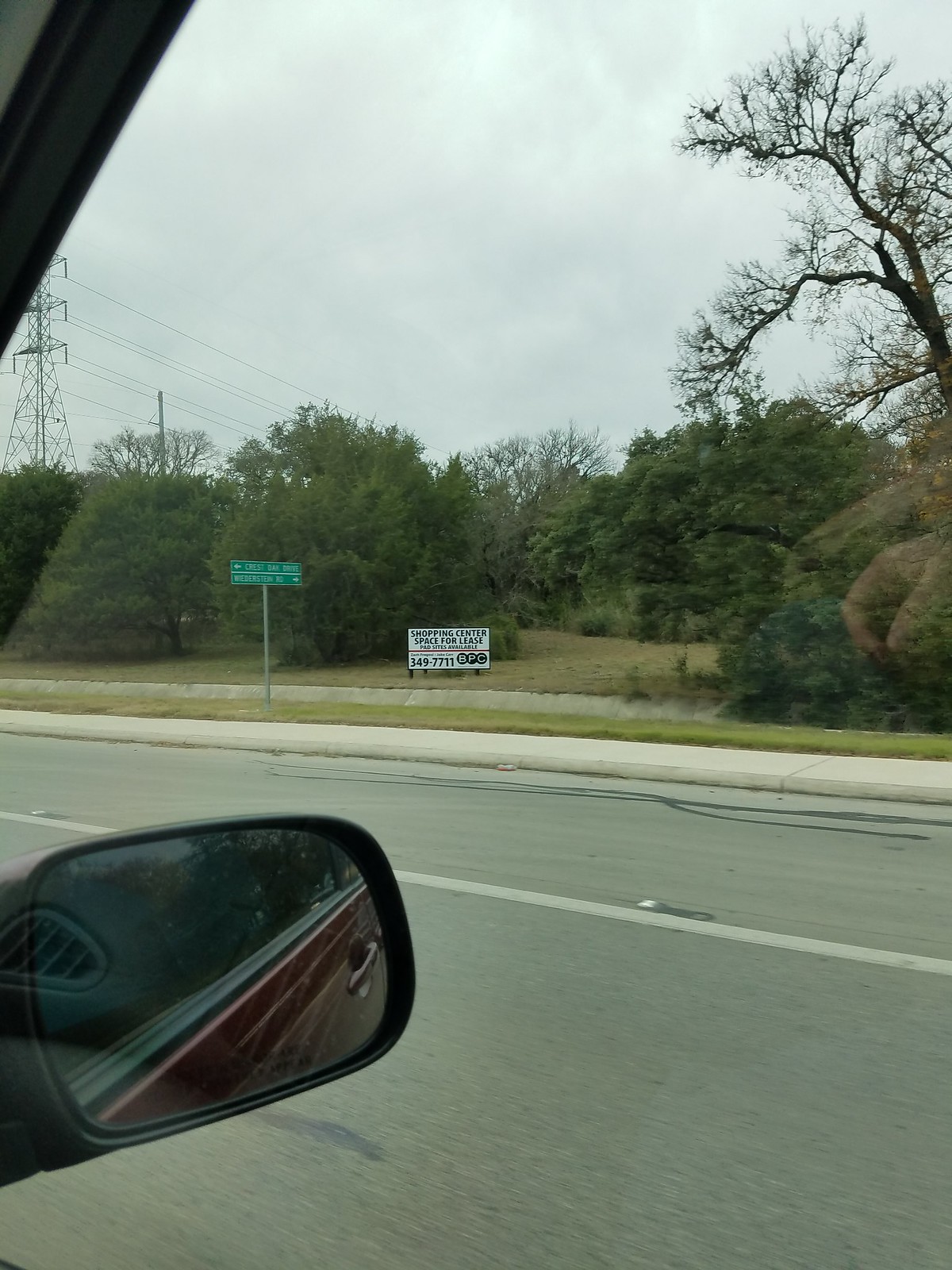In this image, taken from the right side window of a car, the scene gazes out through a slightly translucent, closed window. The car’s rear-view mirror is visible on the window’s left edge, framing the view of a road marked by a white line. In the distance, a green street sign can be seen, though it is too far away to read its inscription. Closer to the foreground, a white sign stands on a grassy patch near a sidewalk, adorned with what appears to be a phone number and words that are not legible. The grassy area is surrounded by numerous trees, adding a sense of depth and natural beauty. On the right-hand side of the image, a leafless tree stands atop a rocky area, creating a stark contrast against the backdrop. Beyond, large power lines stretch across the cloudy sky, adding an industrial element to the otherwise serene landscape.